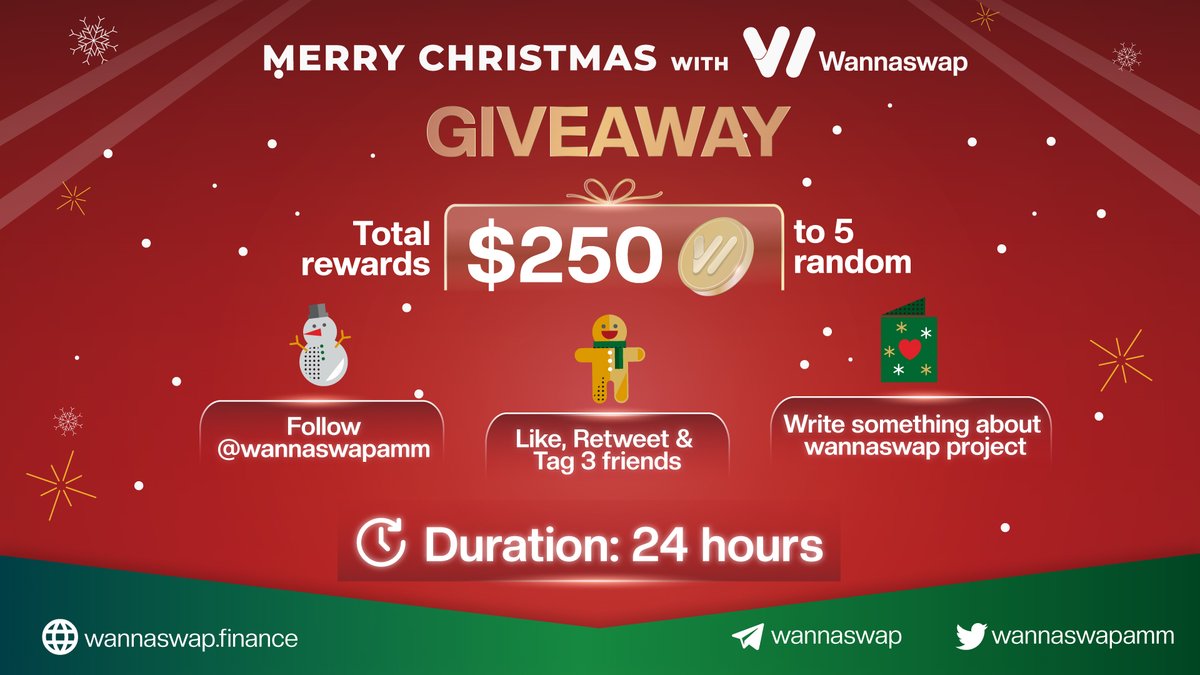The image is a landscape-oriented, Christmas-themed advertisement for WannaSwap, featuring a festive design with a predominantly red background accented with green at the bottom. The backdrop is adorned with scattered snowflakes and white dots representing snow.

At the top of the ad, in bold capital letters, it reads "MERRY CHRISTMAS WITH WannaSwap," with the WannaSwap logo, resembling a 'V' with an additional slash, placed next to it. Below, the word "GIVEAWAY" is prominently displayed in gold, also in all capital letters.

Further down, the ad announces "Total Rewards $250 to 5 random" participants. Adjacent to the "$250" is a gold coin adorned with the WannaSwap logo, highlighted by a line on the left side and a top bow for added festive flair.

The bottom section of the advertisement is divided into three distinct buttons, each accompanied by a specific icon:
1. The left button displays a snowman and reads "Follow @WannaSwap AMM."
2. The center button features a gingerbread man and instructs viewers to "Like, Retweet, and Tag Three Friends."
3. The right button, adorned with a greeting card, encourages users to "Write something about WannaSwap Project."